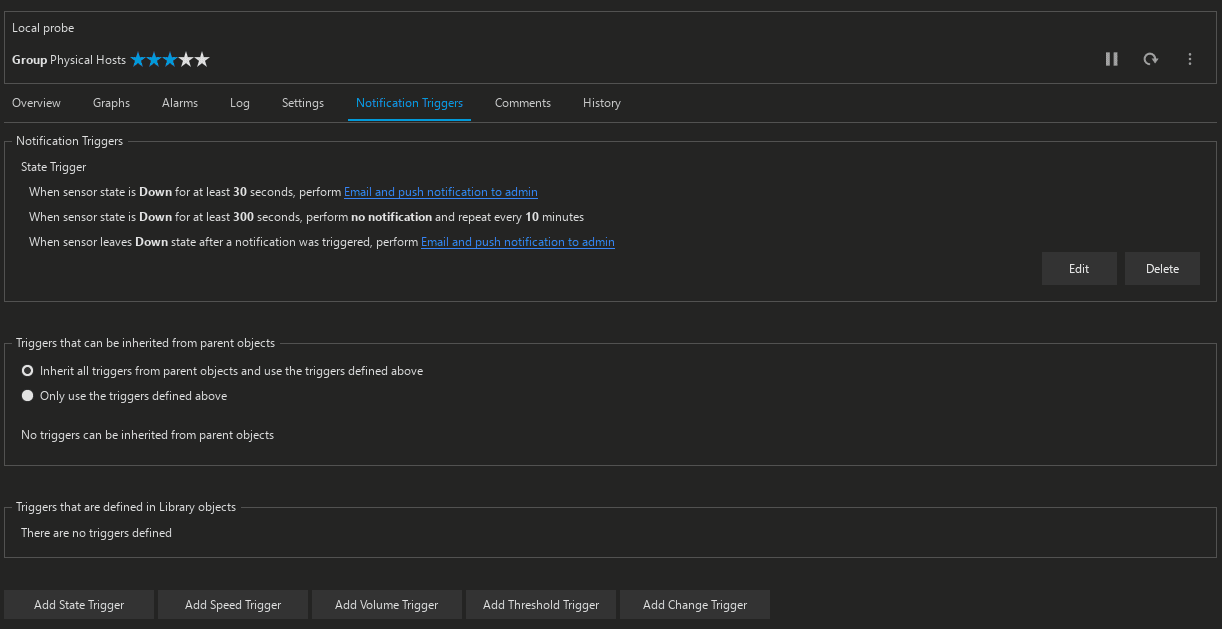This image showcases a user interface of an application displayed in a wide landscape orientation. The interface features a dark gray background with white text and blue accent colors. At the top left corner, a star rating system is visible, showing a rating of three out of five stars. The highlighted stars are blue, whereas the remaining two are white.

Below the star rating is a horizontal menu with clickable tabs for various sections: Overview, Graphs, Alarms, Logs, Settings, Notification Triggers, Comments, and History. The "Notification Triggers" tab is highlighted in blue with a prominent blue underline, indicating it is the selected section.

Within the Notification Triggers section, there are multiple settings related to trigger notifications. These include a section labeled "State Trigger" flanked by three elements that define and limit the trigger settings. An "Edit" button and a "Delete" option are available to the right of these elements, allowing users to modify or remove triggers as needed. Additionally, this area contains blue hyperlinks for further actions.

Further down, there is a subsection titled "Triggers that can be inherited from parent objects," featuring radio buttons to select between two items, each described by a sentence. Below this, another subsection titled "Triggers are defined in library objects" is present.

At the bottom of the interface, there is a row of buttons for adding various types of triggers: "Add State Trigger," "Add Speed Trigger," "Add Volume Trigger," "Add Threshold Trigger," and "Add Change Trigger."